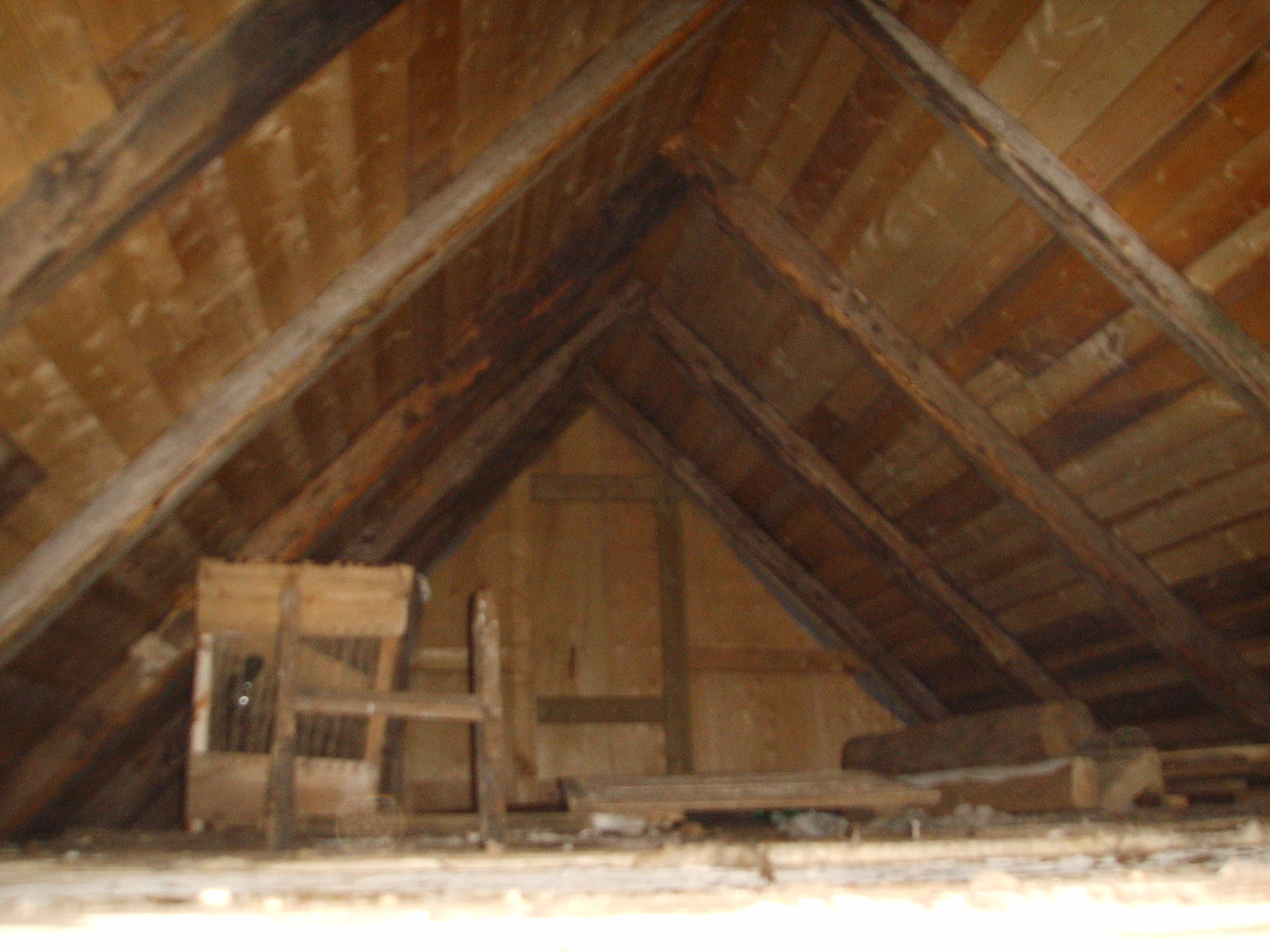The image depicts an interior view of a dilapidated attic space, characterized by its aged wooden construction. The setting is an indoor, dusty attic, with a triangular ceiling made entirely of wood, supported by evenly spaced wooden beams. These beams run parallel to each other and are overlaid with two-by-four planks, extending uniformly along the roof's pitch.

The space appears quite neglected, with a wooden floor in poor condition, and scattered debris that includes possibly broken tables, pieces of furniture, and lumber. The lighting within the attic suggests there are no windows or doors allowing natural light or air to enter. Though one of the far walls vaguely resembles a door shape, emphasizing the old, eerie nature of the setting. The predominant colors in the image are various shades of brown and tan, highlighting the attic's overall wooden and weathered character.